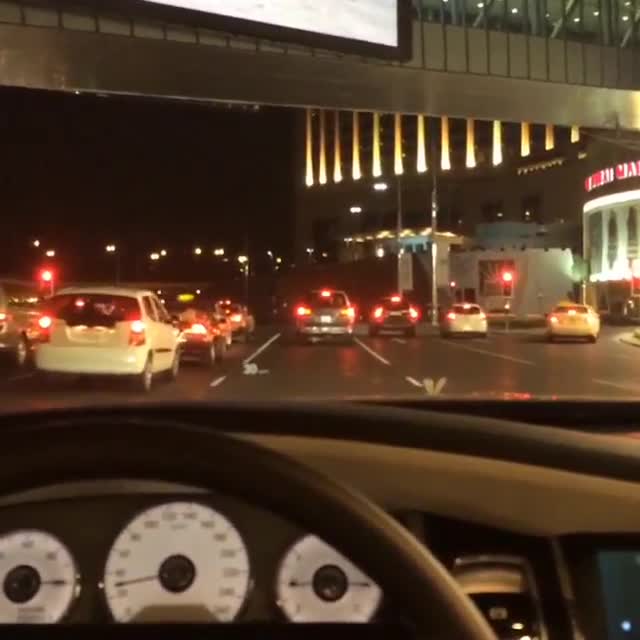This detailed caption describes the scene from the perspective of a driver inside a left-hand drive car at night. The car’s interior features a tan-colored steering wheel and dashboard with three white gauges bearing black numbers, though the precise readings are indistinct. A silver "V" emblem is visible on the car's hood through the windscreen. The exterior view reveals a multi-lane highway crowded with vehicles, all displaying red brake lights possibly due to a traffic light. The lanes to the left and right of the car each contain several cars, with some appearing to make a U-turn or negotiating a roundabout near a building. Above the highway, a glass-enclosed pedestrian walkway with ceiling lights and a white sign is apparent. Additionally, there are illuminated buildings in the distance and overhead street lamps casting light on the scene, contributing to the dark night sky.